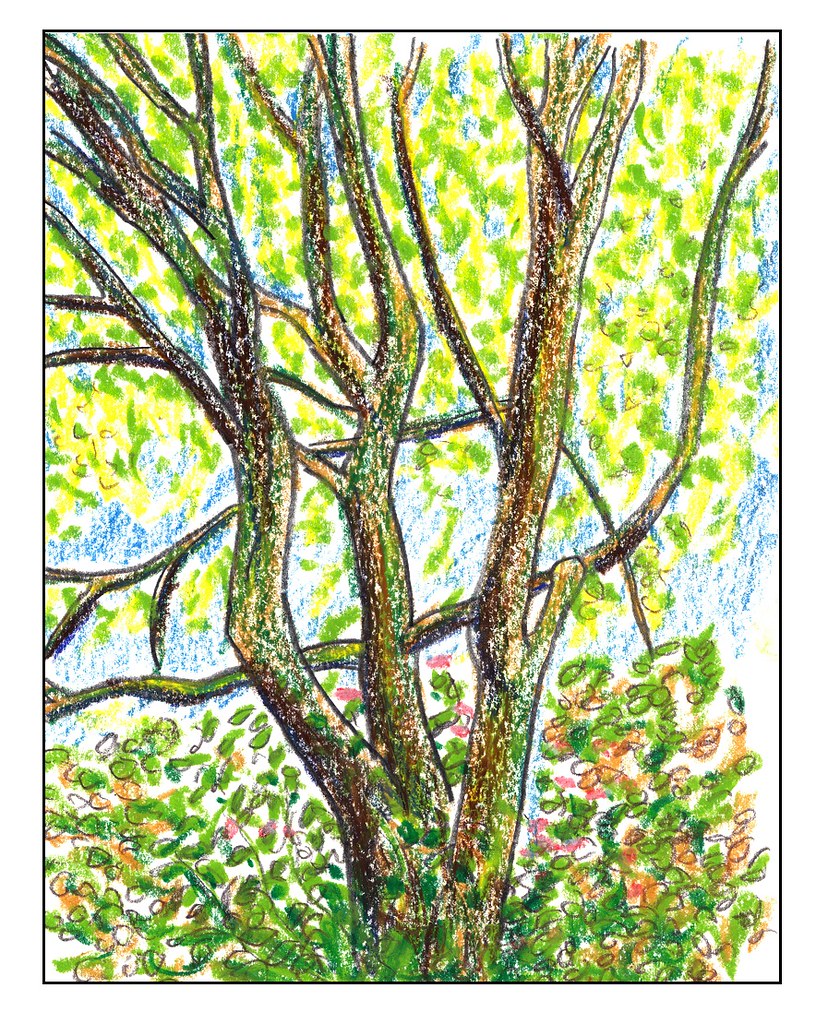This is a colored pencil drawing of a tree, striking in its detailed yet simplistic design. The tree is adorned with a vibrant mix of yellow, green, and orange leaves, some artistically represented as splotches and others meticulously drawn. In one section, the leaves are depicted with colorful patches surrounded by small circles, adding to the abstract nature of the piece. A hint of blue sky peeks through the foliage, while patches of what appears to be moss cling to the tree, enhancing its natural richness. The illustration is set against a standard white paper background, with the white spaces artistically interspersed among the colored areas. Surrounding the entire artwork is a black border, approximately three to four pixels thick, framing the image neatly. Despite the absence of a signature or any credits, this abstract yet recognizable depiction of a tree offers a visually pleasing composition.